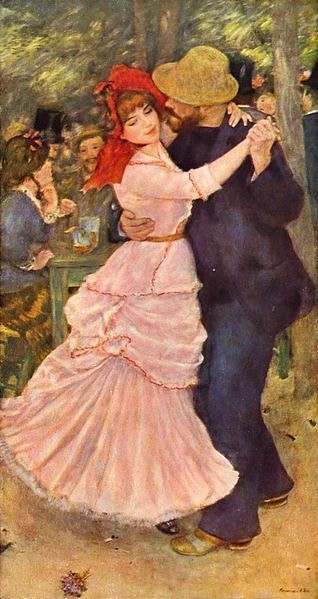The image resembles an Impressionist painting or print, with a vertical orientation, depicting a lively outdoor scene set in the 19th century. Central to the composition are a young couple dancing. The woman, wearing an ankle-length pink dress with frilly layers and a big red bonnet, has blonde hair and exudes youthful prettiness. The man, dressed in a dark blue suit and light brown shoes, sports a straw-colored hat and a brown beard. He holds her waist with one hand and her hand with the other as they dance closely together.

Behind them, under a tree, sits a man and a woman at a green table, laughing and enjoying drinks. The woman in the background wears a blue dress. The setting includes lush green trees and a brown dirt ground, contributing to an atmosphere reminiscent of a cheerful outdoor gathering with people dressed in old Victorian attire, including top hats and mustaches. The painting is rich in detail and captures a moment of joy and connection in a vibrant, historical context.